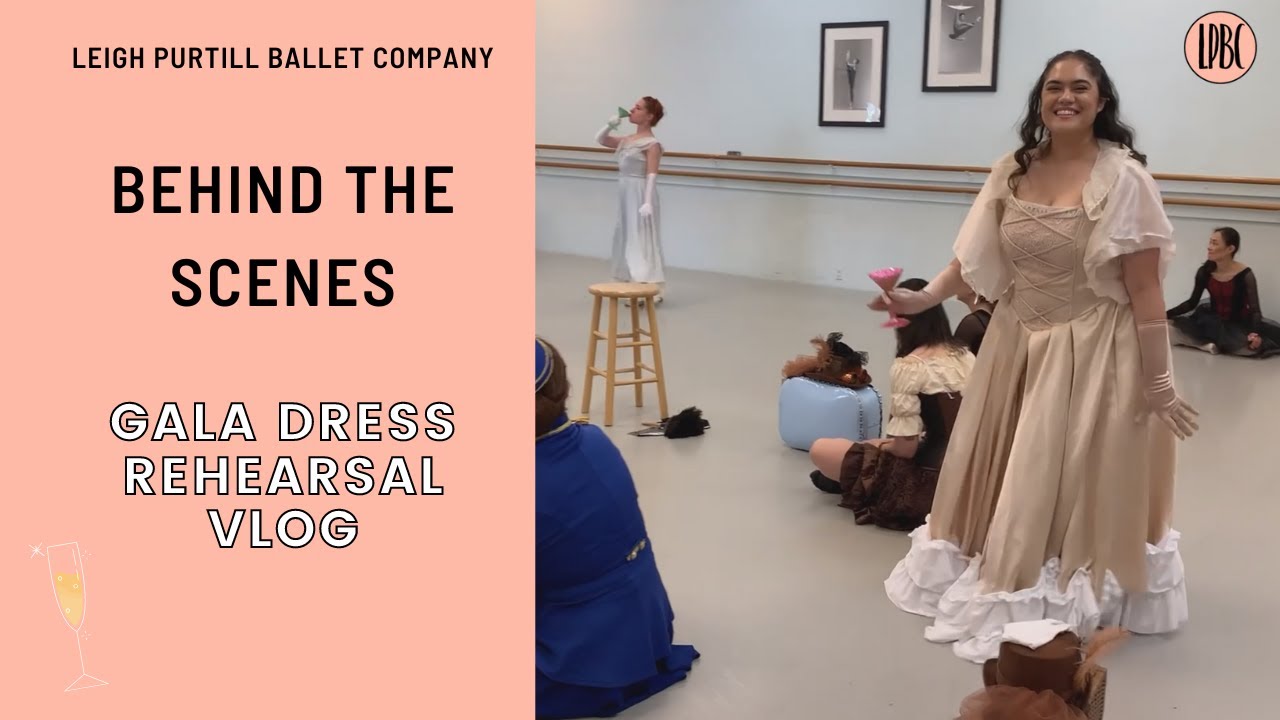The horizontal landscape image is a flyer for the Leigh Purtill Ballet Company, detailing "Behind the Scenes" of their "Gala Dress Rehearsal Vlog." The left third of the image features a pink background with black and white text: at the top, in black, it says "Leigh Purtill Ballet Company," followed by "BEHIND THE SCENES" in larger black font, and finally "GALA DRESS REHEARSAL VLOG" in large white text outlined in black. 

The right side is a vivid snapshot from a ballet studio. The foreground is dominated by a full-figured young woman with long dark wavy hair, attired in a cream and white old-fashioned ball gown featuring flouncy trim at the bottom and on the sleeves. She accessorizes with beige gloves and holds a pink martini glass in her right hand, looking at the camera with a happy grin. The floor is white concrete. Scattered throughout the background are several other people in various costumes, including one person in a white cocktail gown with white gloves and short hair, who appears to be drinking from a glass. There is a bottle of champagne positioned at the bottom left corner of the image. Despite the activity in the room, the focus remains on the smiling woman in the foreground, providing an engaging glimpse into the gala dress rehearsal.